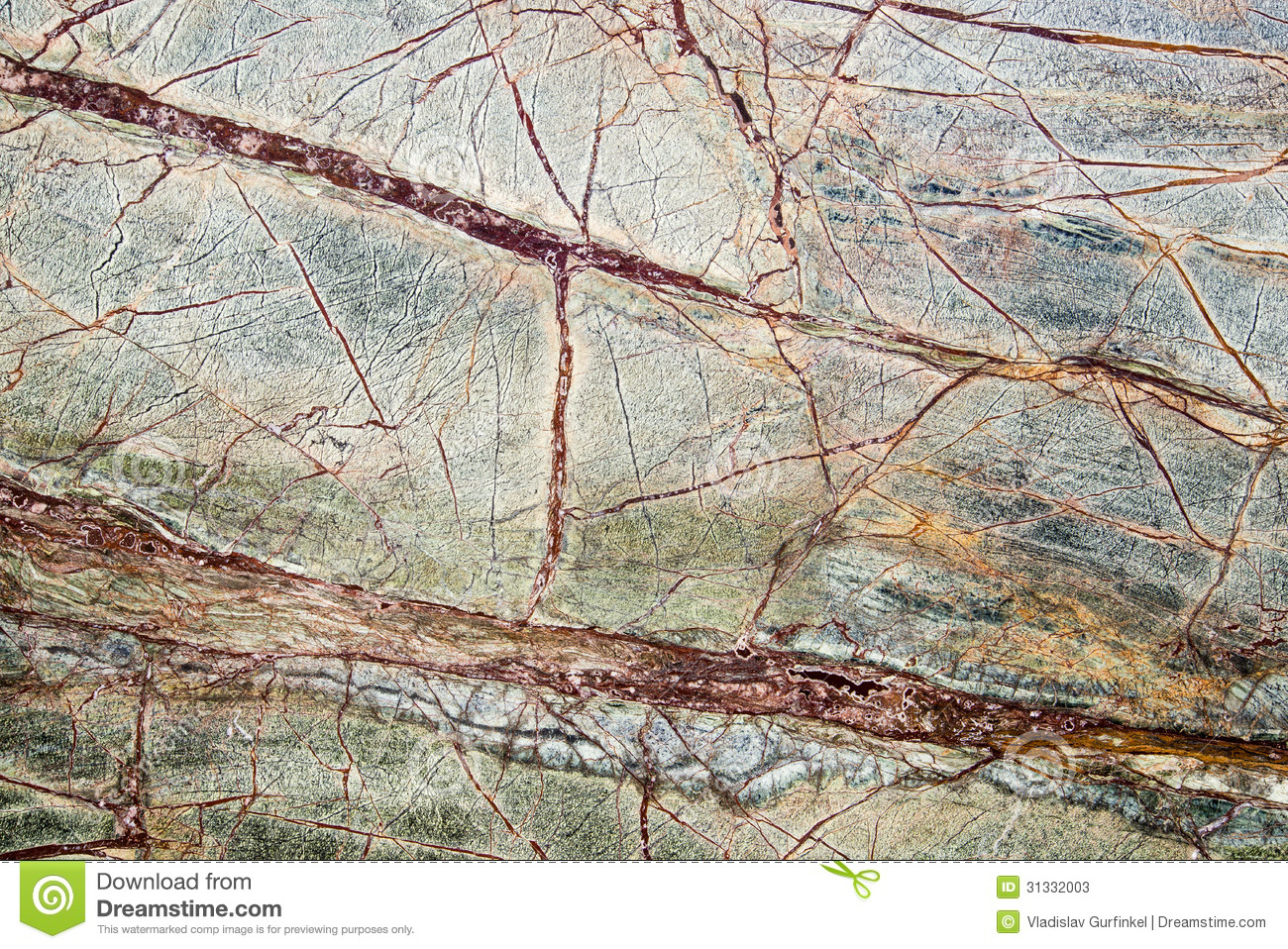The image displays a detailed, highly textured close-up of a very dry leaf, which might also be perceived as intertwining tree branches or veins across rock due to its intricate network. The leaf, primarily colored in shades of light green, darker green, brown, and spots of white, features two prominent horizontal wings extending from left to right, with numerous tiny veins branching off in every direction. These veins are highlighted with a burgundy hue that adds complexity to the pattern. This image, rectangular and horizontally oriented, also includes transparent watermark spirals, contributing to the overall texture.

At the bottom of the image, there is a white bar. On the left side of this bar, a green icon with a downward arrow and spiral is accompanied by the text "download from Dreamstime.com." On the right side are two lines of text: the first line contains the image number "31332003," and below it, "Vladislav Gerfinkel, Dreamstime.com" is listed. The overall composition evokes both the intricate beauty of nature and the meticulous detail of a fine painting.